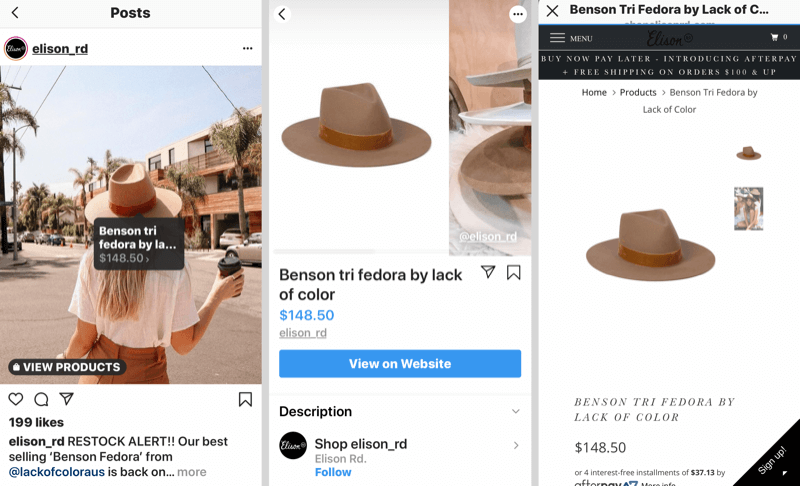The provided voice description captures an Instagram advertisement in detail. Here's a polished and detailed caption based on the information given:

---

**Ellison Road Instagram Promotion Overview**

This series of screenshots illustrates an Instagram post by user Ellison Road, promoting a stylish accessory. 

**Screenshot 1:**
A young woman sporting a trendy outfit is captured walking towards palm trees and a building on a city street. She dons a fashionable white t-shirt, rust-colored pants, and a standout fedora. Her long blonde hair flows underneath the fedora, which is available for purchase through the post. A pop-up, positioned near her hat, reads: "Benson Try Fedora $148.50." By clicking on this, viewers are directed to the purchase link. The post has garnered 199 likes. The caption highlights a restock alert from Ellison Road: "Restock alert! Our best-selling Benson Fedora from Lack of Color is back! Click 'more' for additional details."

**Screenshot 2:**
A direct view of the Benson Try Fedora, with a blue "View on website" button, enabling users to explore this brown fedora further on the linked website.

**Screenshot 3:**
The final screenshot leads to the product page on the website, showcasing the Benson Try Fedora, priced at $148.50 or available for interest-free installments of $37.13 via Afterpay. Additionally, a "Sign Up" option is visible in the top right corner for users interested in receiving updates.

---

This caption effectively condenses and sharpens the original voice description while maintaining comprehensive detail.